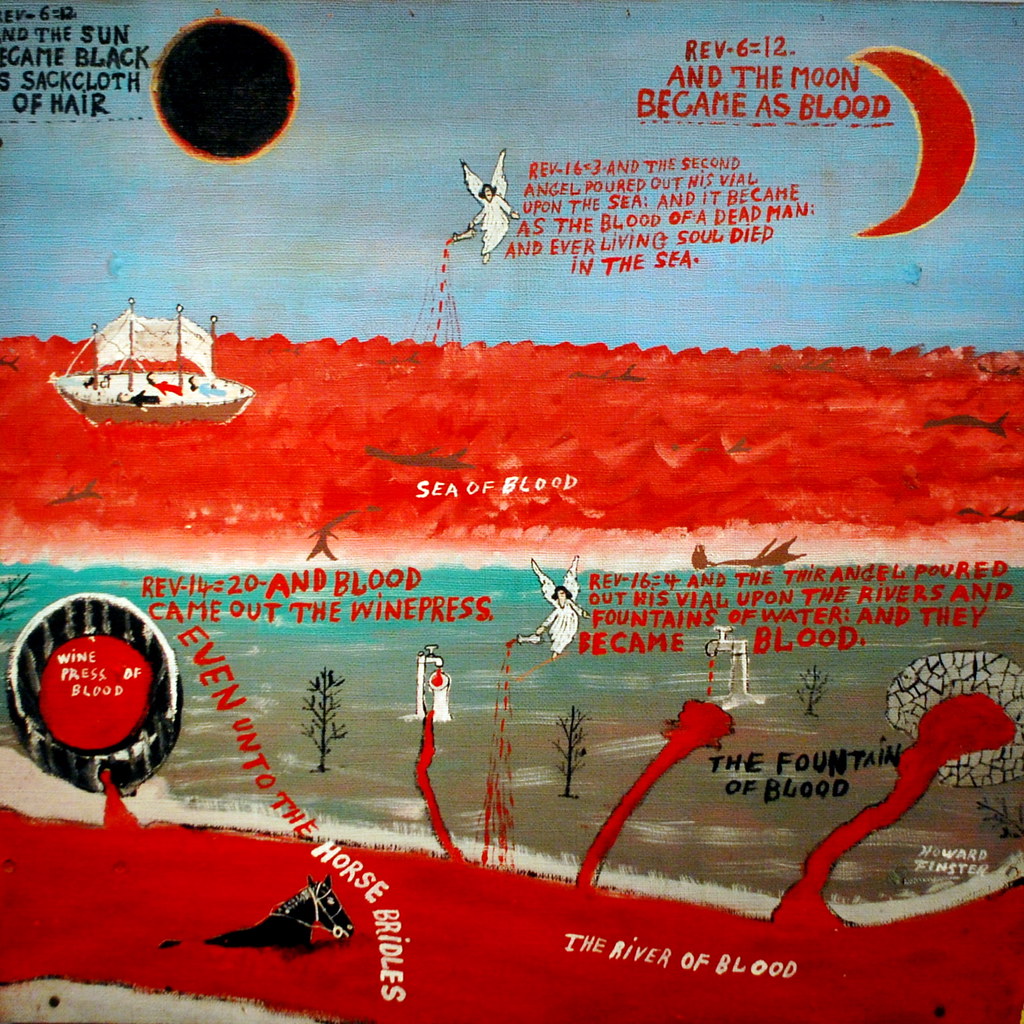The image depicts a large, detailed painting with strong biblical themes. The scene is divided into a red sea and a blue-gray sea. At the top left, a black circle, identified as the sun, with an orange rim, features the text "Rev 6:12 - the sun became black as sackcloth of hair." On the top right, a blood-red crescent moon is labeled with "Rev 6:12 - the moon became as blood." Centered in the image is an angel, hovering above the blood-colored sea, pouring blood from a vial, accompanied by the text "Rev 16:3 - And the second angel poured out his vial upon the sea and it became as the blood of a dead man; and every living soul died in the sea."

To the left of the angel, a small brown sailboat appears adrift in the red sea, with lifeless figures. The sea itself is labeled "Sea of Blood," and it is populated with sea creatures like fish or sharks floating atop. Below this sea, a darker blue-gray sea features additional text and elements. On the bottom left, it reads "Rev 14:20 - And blood came out of the winepress, even unto the horse bridles," next to a circular stone labeled "Winepress of Blood" pouring blood into the sea. On the right, the text "Rev 16:4 - And the third angel poured out his vial upon the rivers and fountains of waters and they became blood" is illustrated by another angel pouring blood into a river.

The bottom right corner of the image contains black text that reads "The Fountain of Blood," set beside a circular fountain with blood flowing out. In the center bottom, a struggling black horse is seen in the river labeled "River of Blood."

Overall, the painting vividly captures apocalyptic scenes described in the Book of Revelation, combining dramatic visual elements and detailed biblical text to convey a powerful narrative.